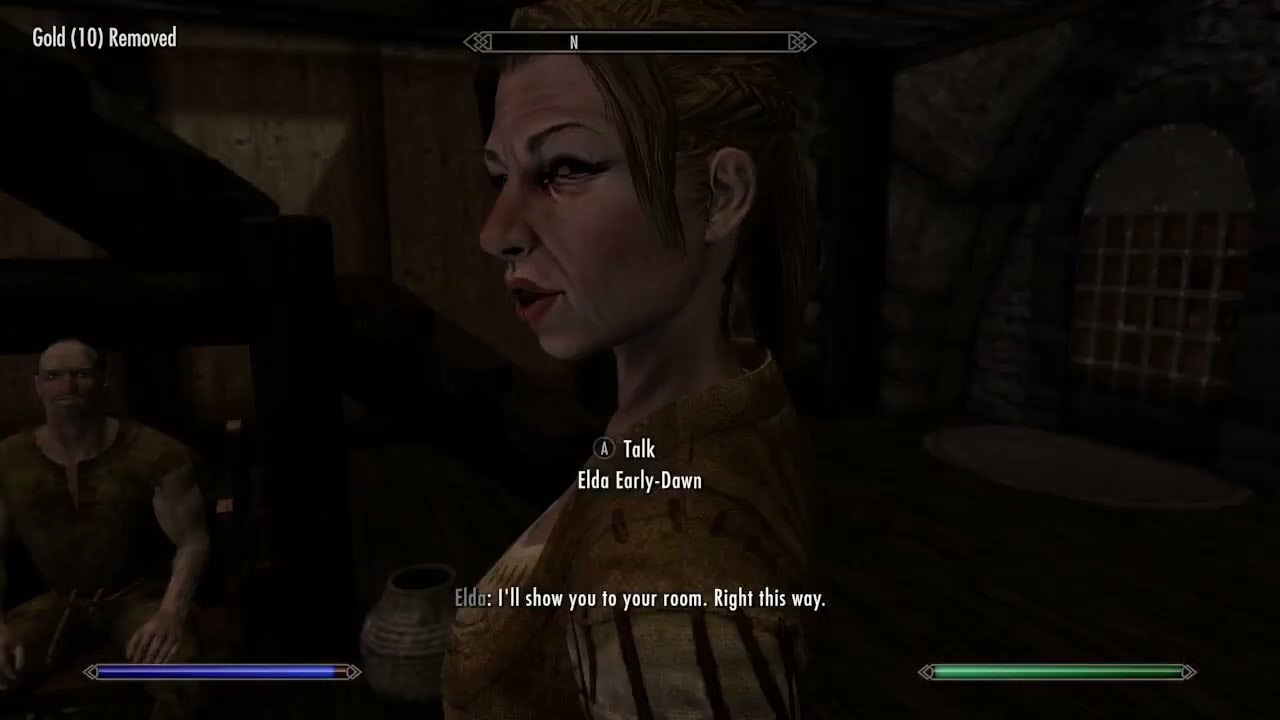The image is a screenshot from an older, role-playing video game, with graphics that appear to be around 10 years old. The primary focus is an older woman named Elda Early-Dawn, characterized by her wrinkled face and tattered clothes, standing slightly angled to the left with her left side facing the camera. She is speaking, and at the bottom of the screen, subtitles clearly display her name and dialogue: "I'll show you to your room right this way." The environment is dark, resembling nighttime, and is possibly set in a medieval-themed inn or tavern. In the background, there's a medieval-styled building, and nearby is a bald, muscular man wearing a green tunic, who seems to be gazing in the viewer's direction. The game's graphical user interface includes two energy bars in the bottom corners—the left is blue and partially depleted, while the right is green and full. The top left corner shows "GOLD 10 REMOVED," and a horizontal compass indicating 'N' is present. Additionally, the screen features action text centered at the top, indicating the player can "TALK" with the button labeled "A."